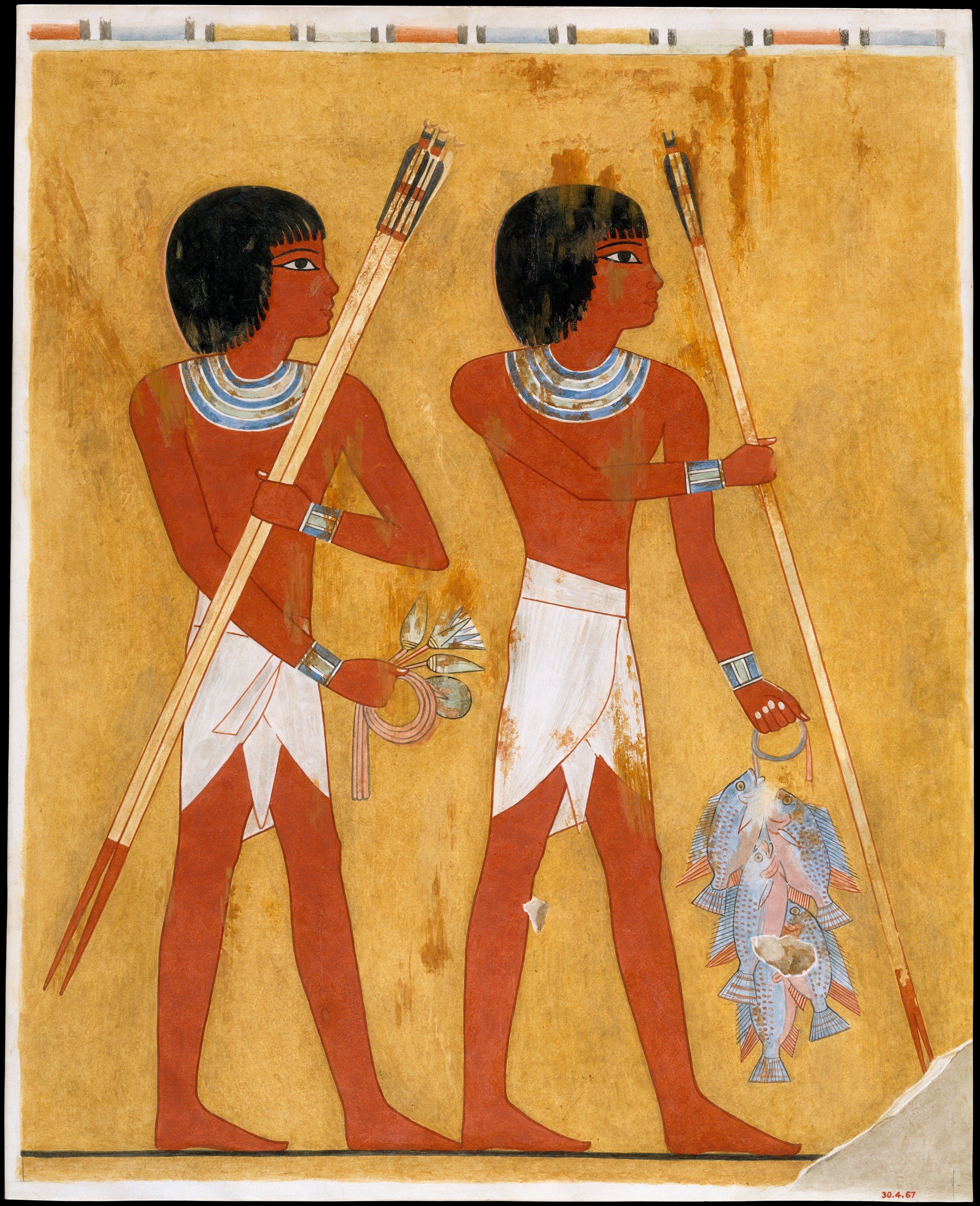This image is a detailed depiction of an ancient Egyptian drawing against a faded scroll or pyramid-like background. It shows two Egyptian men, both with shoulder-length dark hair and black bangs, standing next to a brown wall. They are dressed in traditional Egyptian attire—short white loincloths or skirts with no shirts, adorned only with necklaces. Each man holds a spear in his left hand. The man in the front also carries a rope with four fish hooked to it, while the other holds additional, smaller spears or possibly wires. They both appear to be foraging or engaged in some form of fishing activity. The image includes a numerical inscription at the bottom—30.4.67—and the bottom right corner of the painting appears torn and missing.